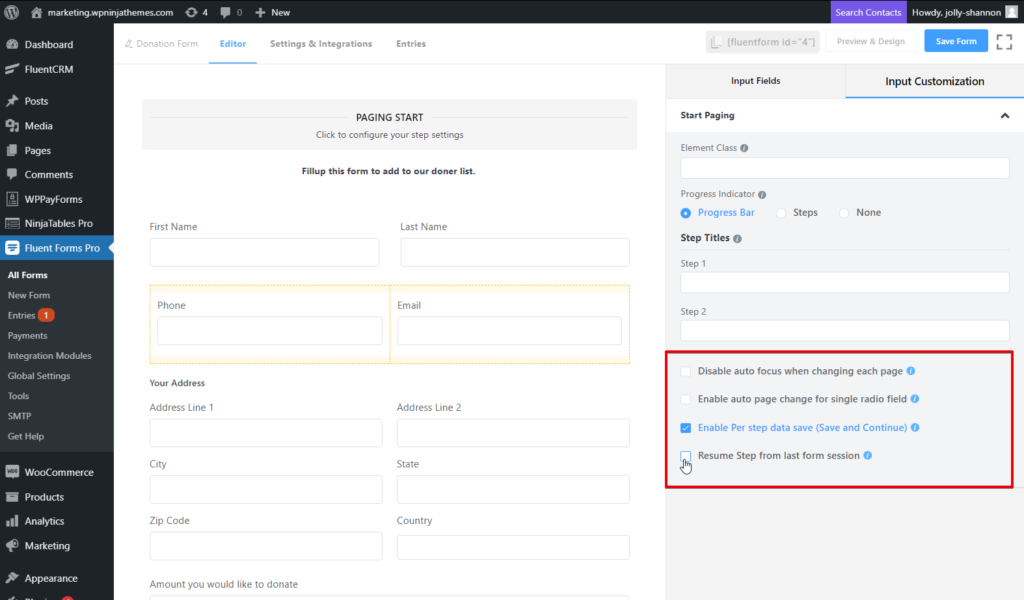This image depicts the interface of an input screen on a wiki site, specifically Wikipedia. In the upper left corner, the Wikipedia logo is prominently displayed—a white circle with a distinct black "W" inside it. Adjacent to the logo, there is a slim navigation bar containing various small, informative elements. Highlighted within this bar is a search feature, clearly marked with the option to "search contacts."

On the left side of the screen, a dark black rectangular sidebar extends vertically, serving as the main menu for the site. This sidebar is filled with hyperlinks, providing access to numerous sections of the wiki. These hyperlinks facilitate the navigation and exploration of the site's extensive content.

The central portion of the screen is dedicated to data entry fields, where users can input information such as name, address, zip code, and country. To the right of this main input section, additional input fields and customization options are available, allowing users to modify and personalize the information they enter. This image provides a comprehensive view of the input and navigation features on this particular wiki site.